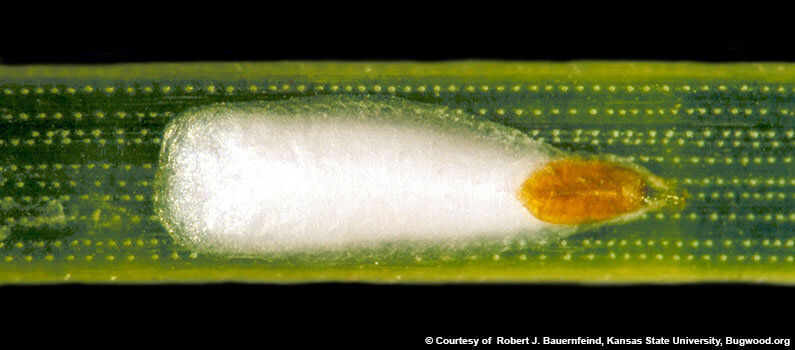This image, set against a green background with black borders at the top and bottom, appears to be a detailed photograph of a green leaf, possibly from a banana tree. The leaf is characterized by yellow borders along the top and bottom edges, along with neat rows of yellow dots that could represent either natural patterns or scientific markers. In the middle of the leaf, there is a white, slimy trail indicating the recent passage of a bug. This bug, located near the front of the trail, has an orange, somewhat translucent body with tucked-in wings and a little black head. Additional text at the bottom right corner credits Robert J. Barnfriend from Kansas State University and bugwood.org for the image. The photograph is finely detailed, capturing the intricate textures and colors of the leaf and its small inhabitant, and might be a microscopy photo based on its highly magnified appearance and meticulous structure.